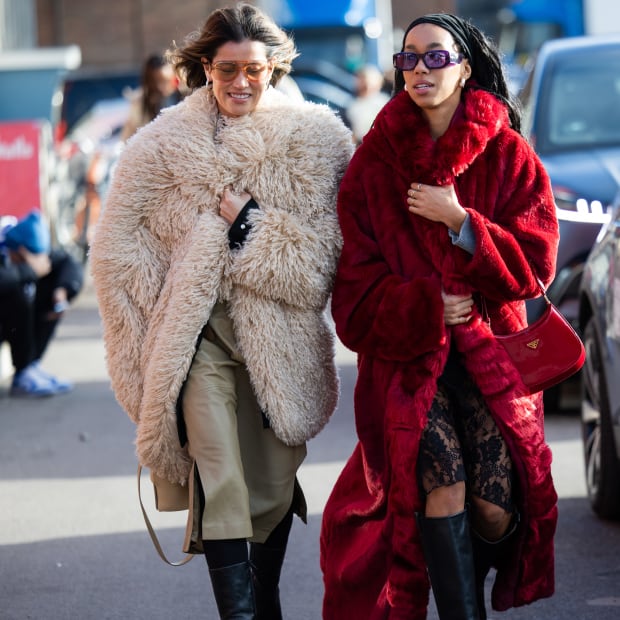The image captures two women walking together on a busy, cold, and somewhat windy street during the day. Both are dressed warmly in thick coats and sunglasses. The woman on the left is white with long brown hair blowing in the wind. She sports a small smile and wears light-colored, possibly amber-tinted sunglasses. Her attire includes a knee-length, woolly, cream-colored coat that she holds shut with her right hand, and she pairs it with khaki-colored pants and black knee-high boots.

To her right, the black woman, with a headscarf or headband around her head, is wearing black glasses with a purple tint. Her striking red, furry coat extends nearly to the ground, revealing just the bottom of her lacy black dress and knee-high black boots. She also carries a red purse. The setting indicates a bustling street with blurred figures of pedestrians and parked cars, emphasizing the everyday urban environment.